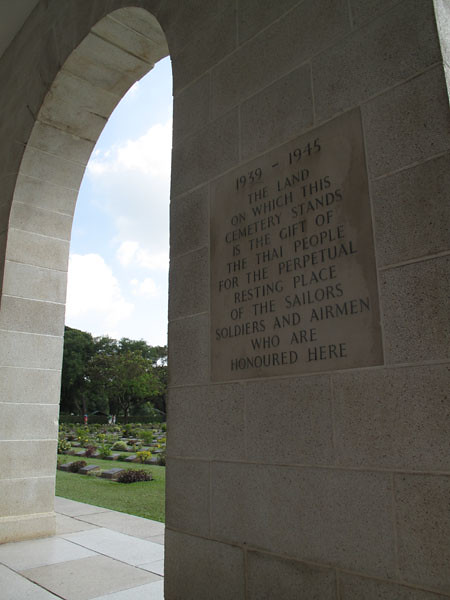The image features a detailed view of a cinder block wall on the left with an open-air archway at its center, topped by a rounded arch. Within this archway, a smooth stone plaque is embedded, inscribed with the dedication: "1939-1945. The land on which this cemetery stands is the gift of the Thai people for the perpetual resting place of the sailors, soldiers, and airmen who are honored here." The gray plaque seamlessly blends with the wall's coloration. Through the archway, a meticulously maintained cemetery stretches out, characterized by rows of headstones interspersed with vibrant flower blooms in purple, yellow, and green. The cemetery features a backdrop of lush green trees and is framed by a cloudy sky with patches of blue. The entire scene evokes a sense of solemn beauty, combining the tranquility of a garden with the reverence of a military memorial.